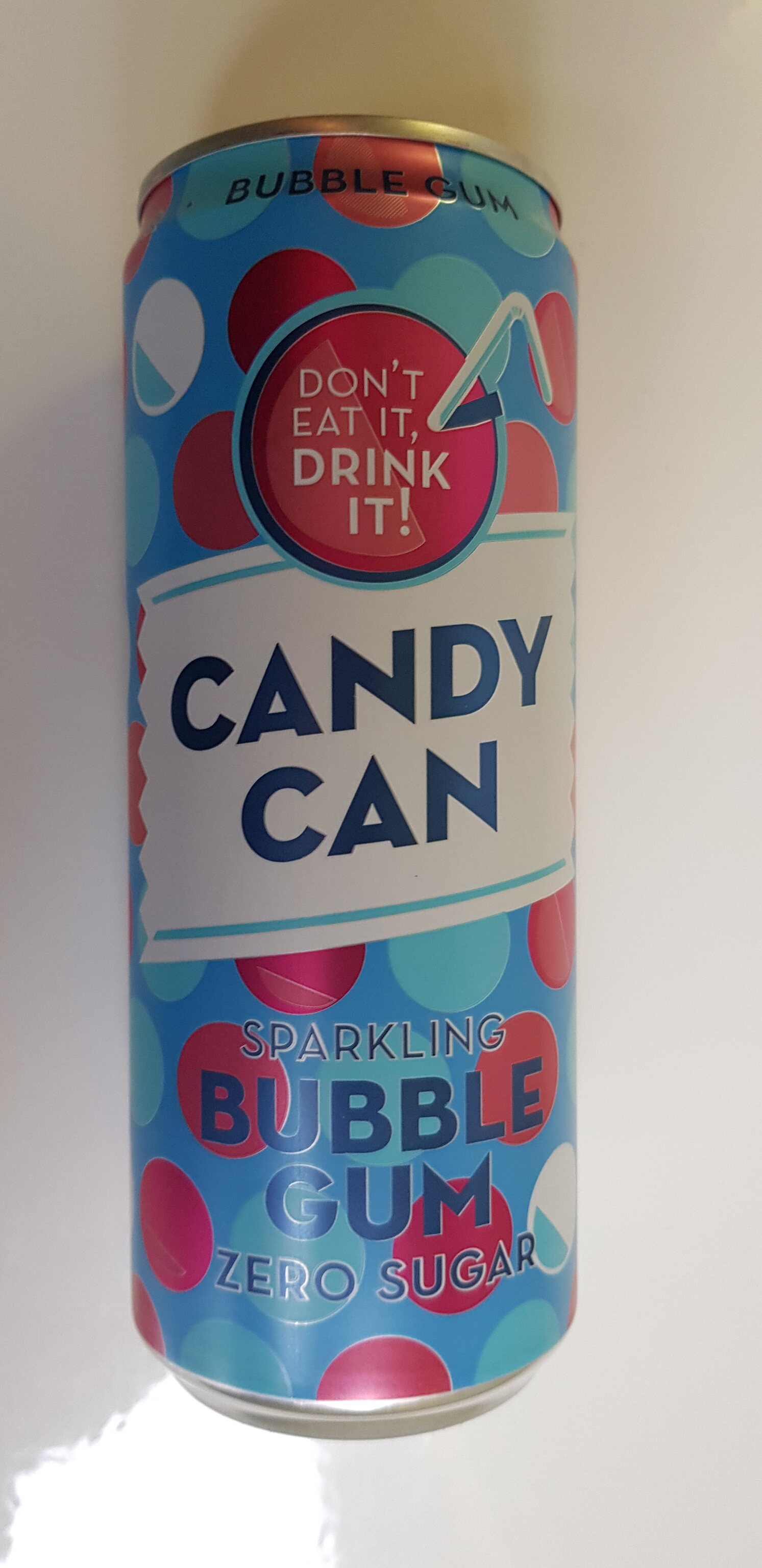This image, set against a grey background, features a vibrant can of sparkling water. The can itself is predominantly blue and is embellished with an array of red and blue dots, interspersed with a few white dots that contain small teal blue semicircles. The label at the top proudly displays the words "Bubble Gum." Below this, a red circle with a straw protruding from it mimics the appearance of looking down into a cup, playfully suggesting the beverage's refreshing nature. A quirky slogan, "Don't eat it, drink it," adds a touch of humor to the design. Further down, a small banner reads "Candy Can," and beneath it, the description "Sparkling Bubble Gum, Zero Sugar" emphasizes the unique flavor and health-conscious aspect of the drink.